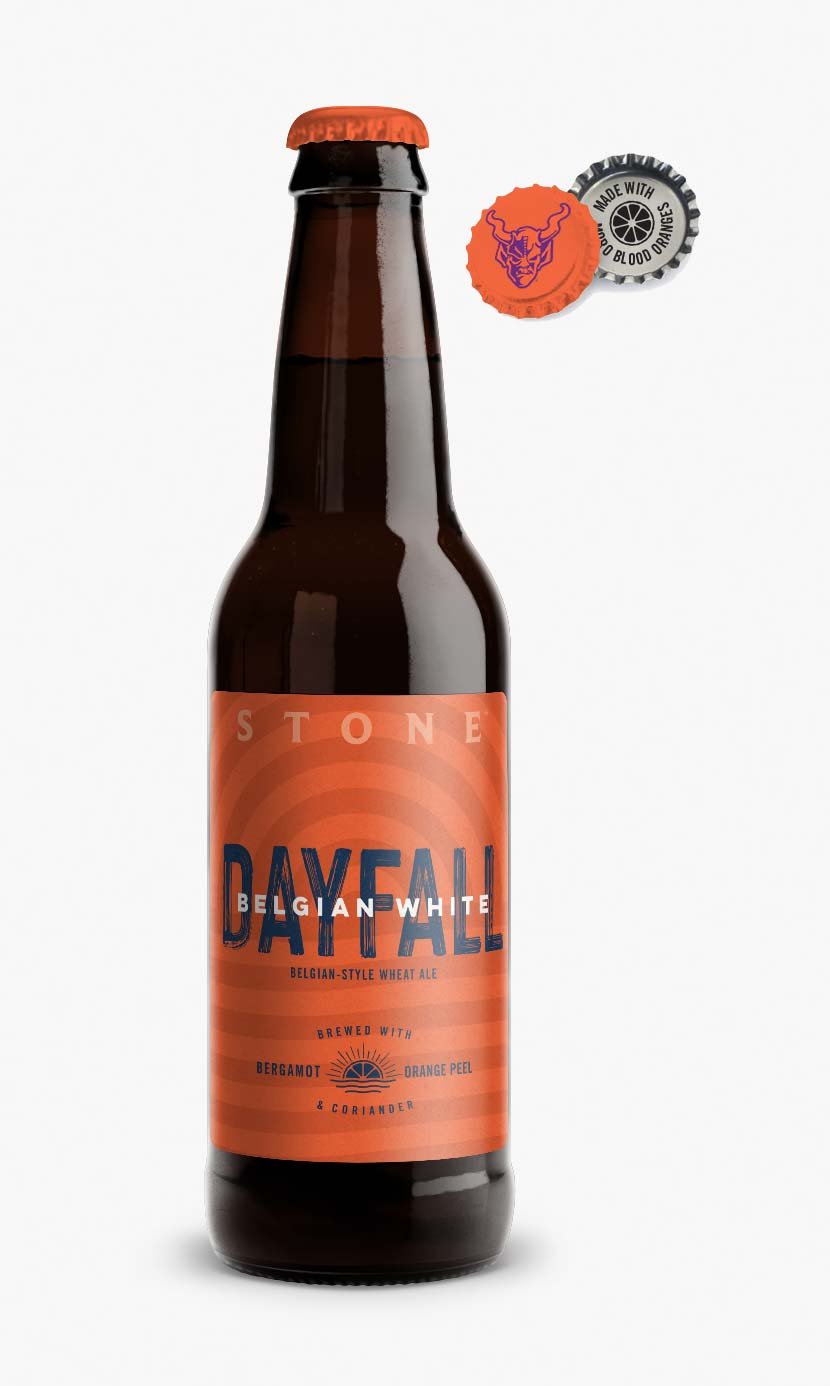The image depicts an advertisement for a craft beer called "Dayfall Belgian White Wheat Ale" by the brewery Stone. The dark brown, standard-sized beer bottle features a vivid orange label displaying the name "Stone" at the top, followed by "Belgian White" and bold blue text "Dayfall." The label also mentions that the beer is brewed with bergamot, orange peel, and coriander, with a graphic of a half blood orange and sun rays. The bottle cap, which is also orange, sports an intricate devil motif in blue. Inside the cap, text confirms that the beer is made with real blood oranges. The image focuses on the bottle, its detailed label, and the unique cap design, emphasizing its artisanal and imported qualities.